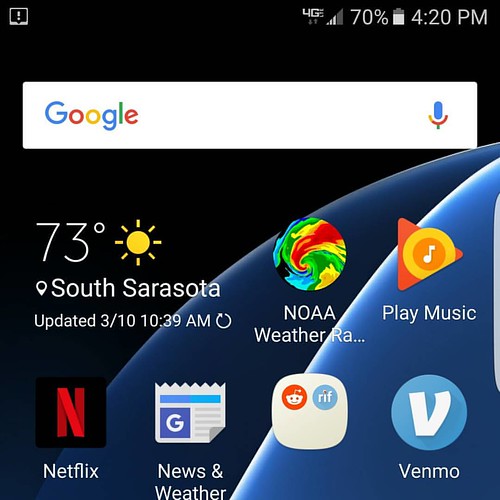The screenshot captures the homepage of a mobile device, though the specific model remains unidentified. At the top of the screen, there is a Google search bar for entering search terms. The homepage prominently showcases several apps, including Venmo, Netflix, Play Music, News and Weather, along with another weather app. The device provides locale information, identifying the location as South Sarasota. The weather data was last updated on March 10th at 10:39 AM, describing it as sunny with a temperature of 73 degrees Fahrenheit. Additionally, the current time displayed on the screenshot is 4:20 PM.